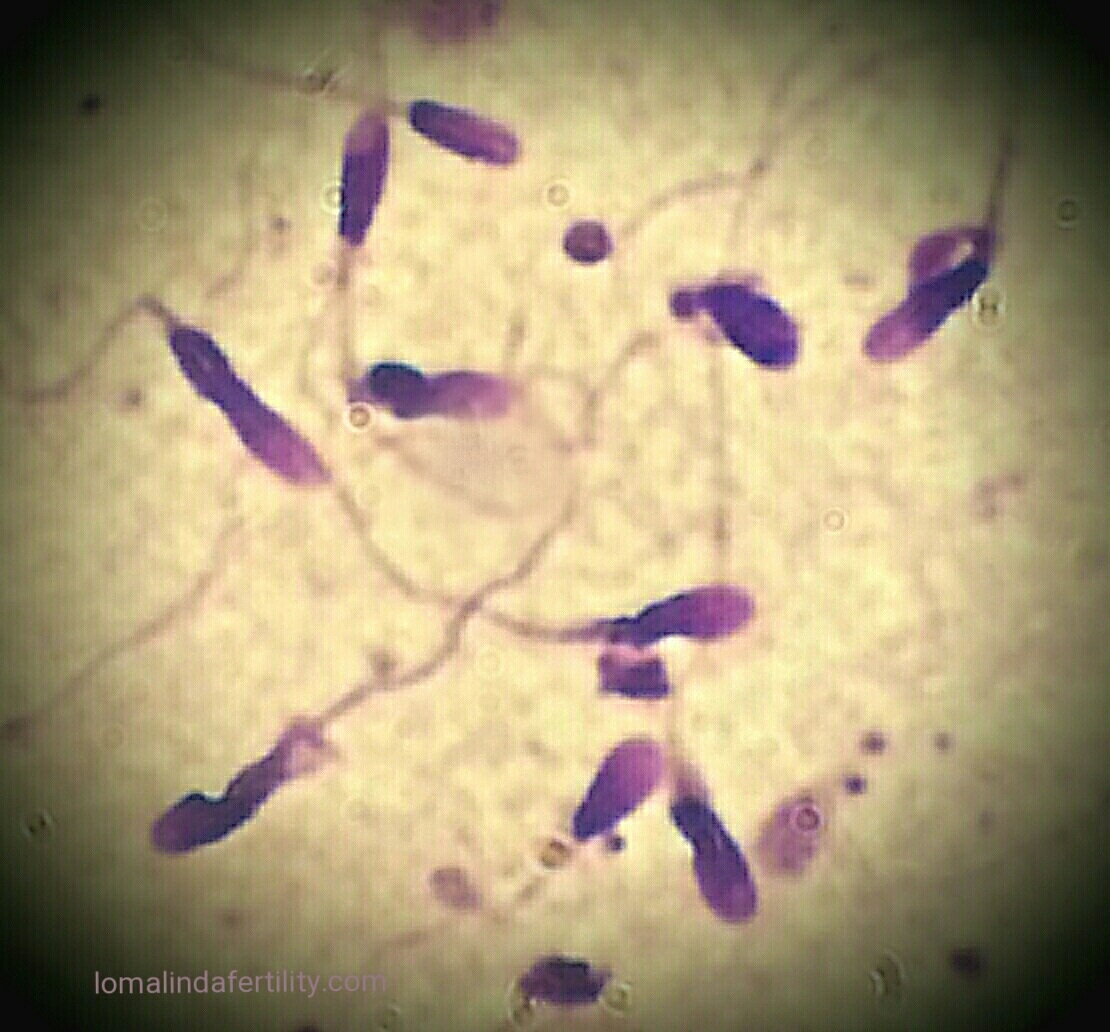This highly magnified image, likely captured through a microscope, depicts approximately a dozen or more elongated spermatozoa swimming through a fluid medium. The sperm cells display a distinctive coloration, with deep purple bodies that become lighter towards their tips. The background is predominantly yellow, possibly due to the microscopy lighting, and is encircled by dark shadowy areas suggesting the microscope's lens edges. Each sperm is characterized by a long, tapering tail, further emphasized by the purple hues. In the bottom left corner, a URL is visible in gray text, reading "llama.lindafertility.com," though the image quality is notably compressed with visible JPEG artifacts. This image seems to be from a fertility study, as indicated by the website reference.